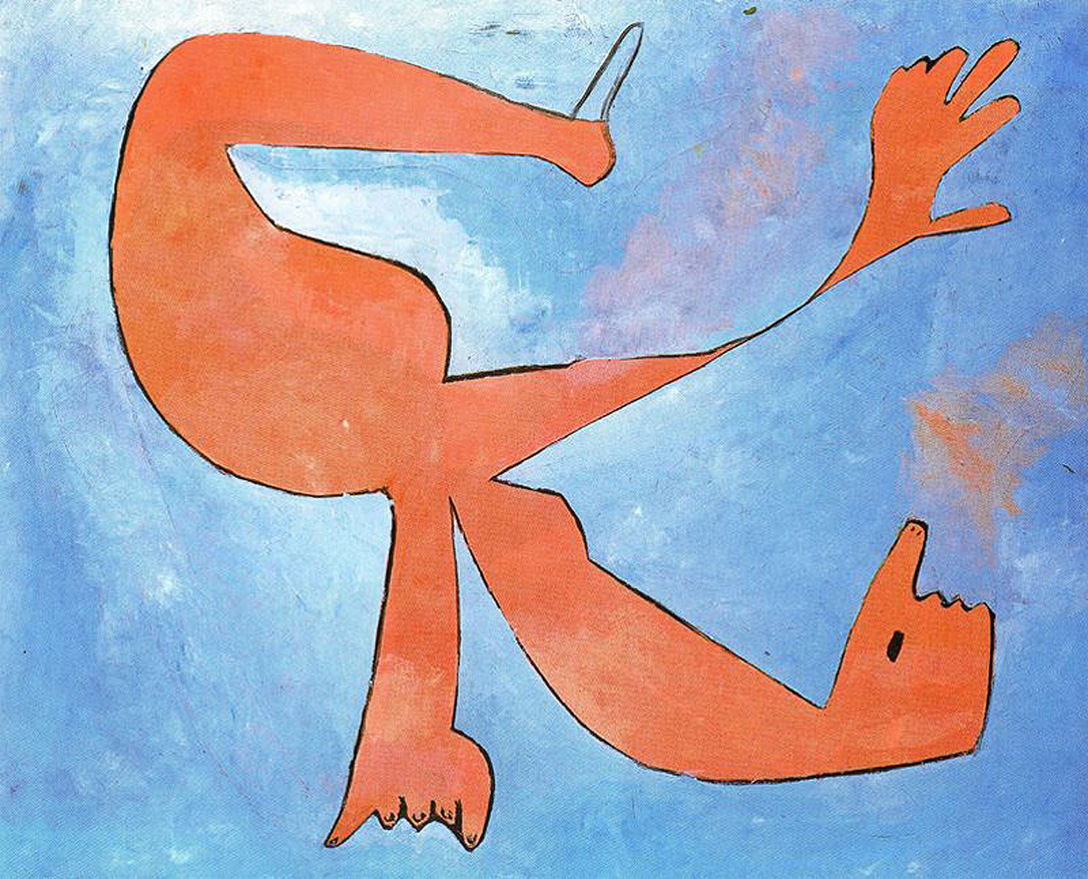In this abstract painting, the background is a mottled mix of light to medium blue with patches of purple, orange, and white. Central to the composition is a unique, somewhat indeterminate figure rendered in orangey-red hues and outlined in black. This figure, perhaps one-dimensional or two-dimensional, encompasses various intriguing features: it possesses a tubular appendage extending from the top, bending leftward and widening into a rounded shape before branching into three distinct limbs. The lower limb, suggesting an arm, terminates in five short, finger-like protrusions. The middle limb stretches diagonally to the right, tapering into a pointed tip with a black dot at the end. The upper limb becomes a thin string that opens into six finger-like extensions of varying lengths. An additional orange splotch decorates the area above and to the right of this appendage, further contributing to the painting's dynamic and whimsical character.